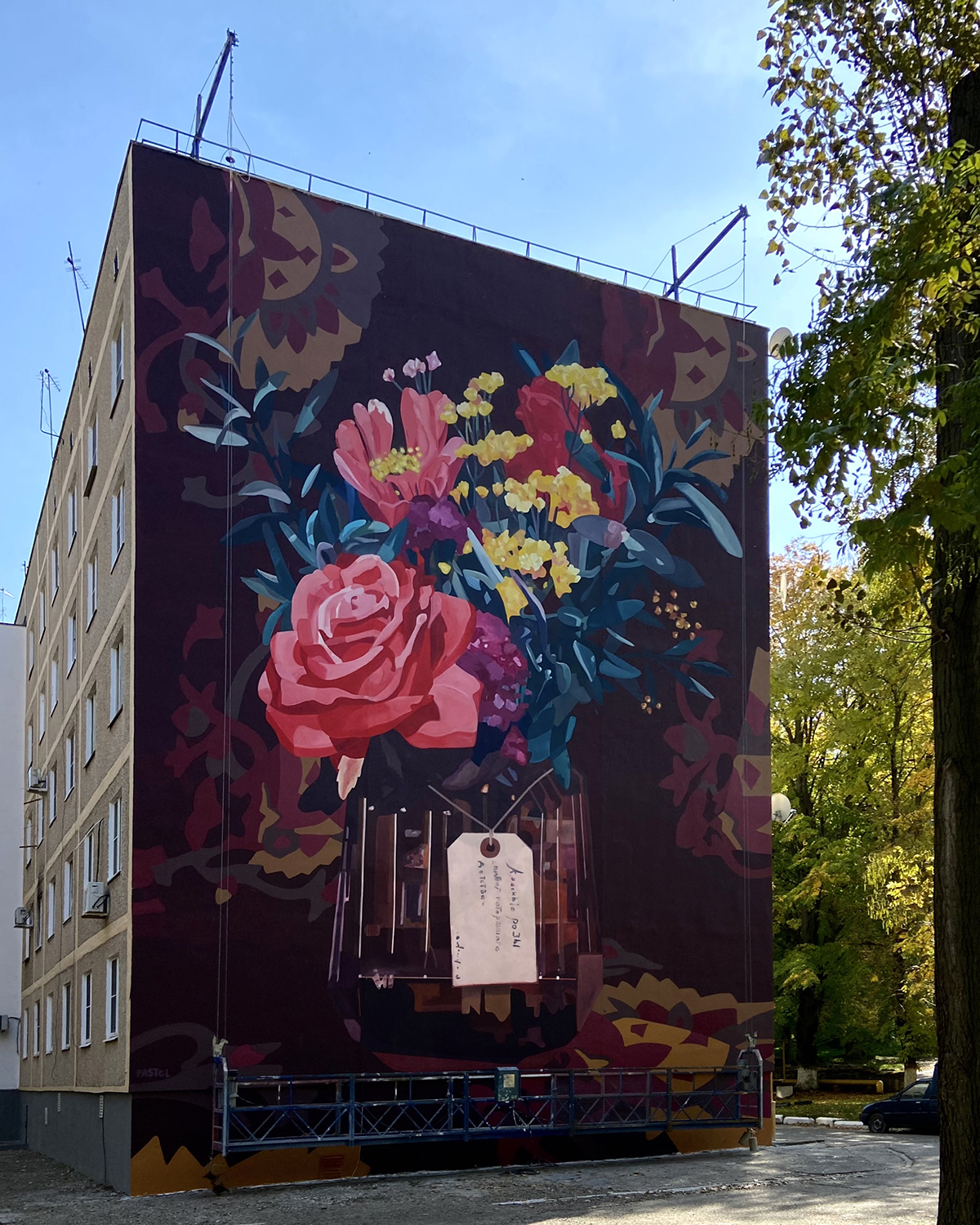The image depicts a vibrant mural painted on the side of a large building, which appears to be between five to six stories high. The side wall of the building, void of any windows, serves as the canvas for this detailed and colorful artwork. 

The centerpiece of the mural is a large bouquet of flowers within a vase, prominently featuring a variety of flora, including pink and purple roses, smaller purple flowers, green leaves, tiny yellow buds, and sprigs of white baby's breath at the top. Attached to the vase is a beige or white tag with sideways lettering. 

The background of the mural bursts with bright colors, predominantly purples and blues, contrasting strikingly against the detailed botanical elements. Surrounding the bouquet are abstract designs that add an additional layer of artistic depth. 

Hanging in front of the mural from the roof is scaffolding that spans the width of the building, supported by cables and placed just below the vase. This structure suggests ongoing work or the recent completion of the mural, further adding to the dynamic nature of the scene.